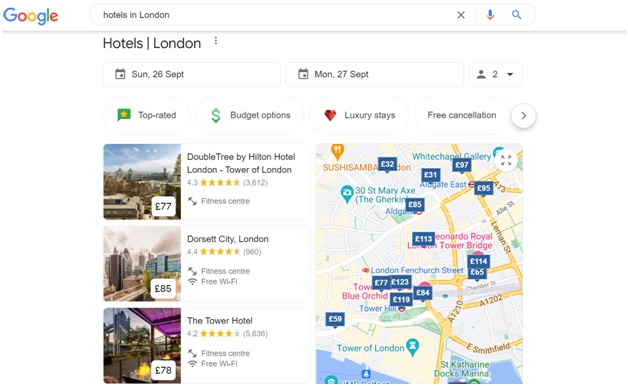A person performed a search for hotels in London, setting their stay from Sunday, September 26th to Monday, September 27th, for two adults. The search results show three specific hotel listings on the left, all priced under £100: the DoubleTree, Dorset City London, and the Tower Hotel. These results are displayed alongside a map on the right, which pinpoints numerous other hotel options. Some map-listed hotels exceed £100, with the most expensive being £123. The map also highlights key landmarks including the Tower of London, Tower Bridge, and the Whitechapel Gallery. No filters such as top-rated, budget, luxury, or free cancellation have been applied yet.